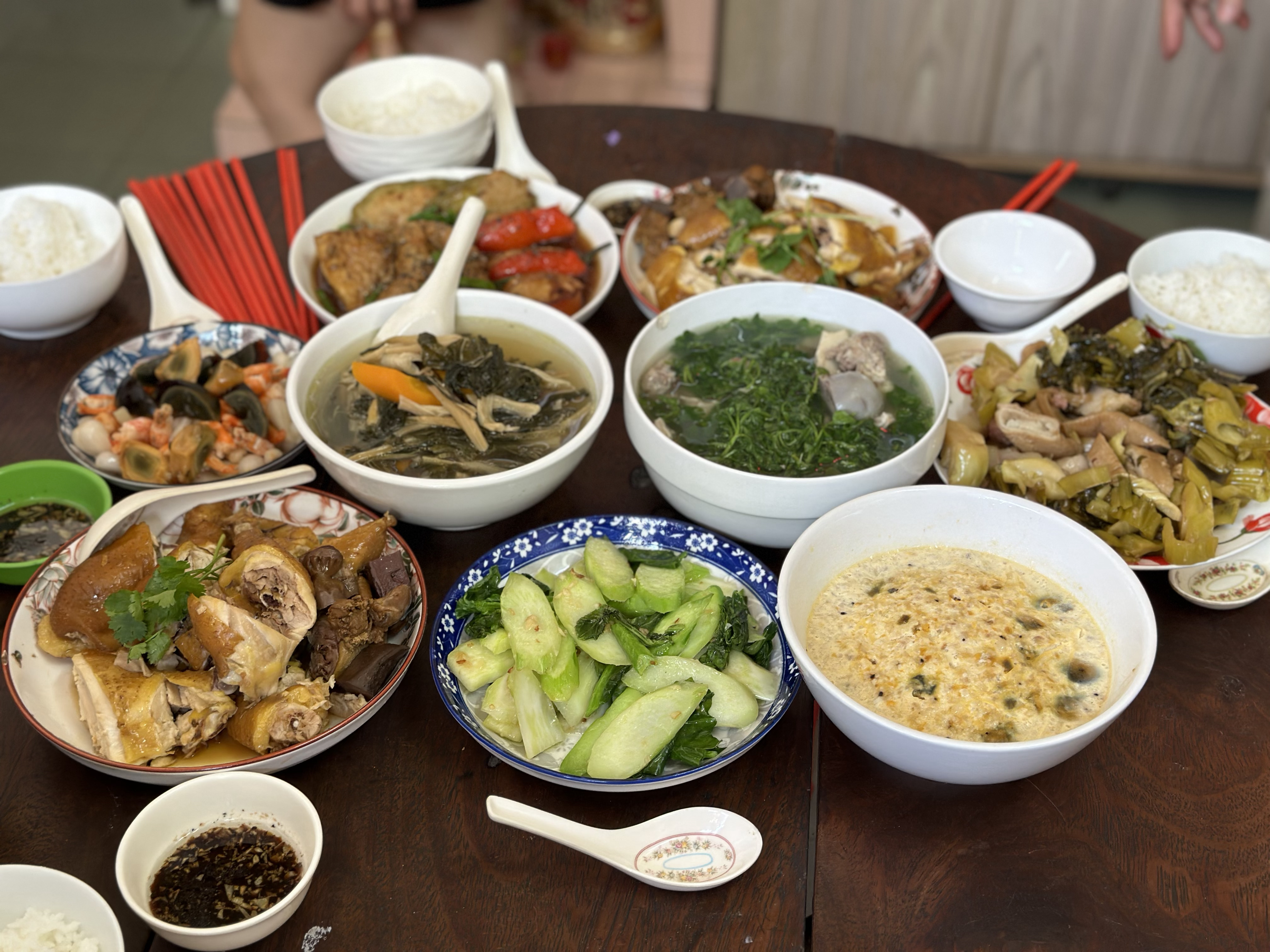The photograph captures a bustling, round, dark wooden table, heavily laden with an assortment of dishes that suggest a large family gathering. Although the entire table isn't visible, we can see an array of 14 plates and bowls presenting a vibrant spread of Asian cuisine. To the far left, a white bowl stands next to a big, wide soup spoon, typically used in Asian countries. Nearby, a bunch of red sticks, likely chopsticks or straws, are positioned alongside other bowls of rice and various plates of food. Prominently in the front, a blue-trimmed plate is brimming with green items, possibly vegetables. Adjacent to it, a mostly white plate features dark reddish-brown accents, filled with meat-based foods enclosed in wrappers. The table also includes soup ladles, chopsticks, and several ornamental and soup bowls, possibly for dishes like dim sum or pot stickers. Visible in the background are parts of two people's legs and hands, hinting at their imminent participation in this substantial, communal meal. Overall, the table presents a dynamic and diverse feast, filled with vegetables, meats, soups, and rice, indicating a hearty meal ready to be shared.